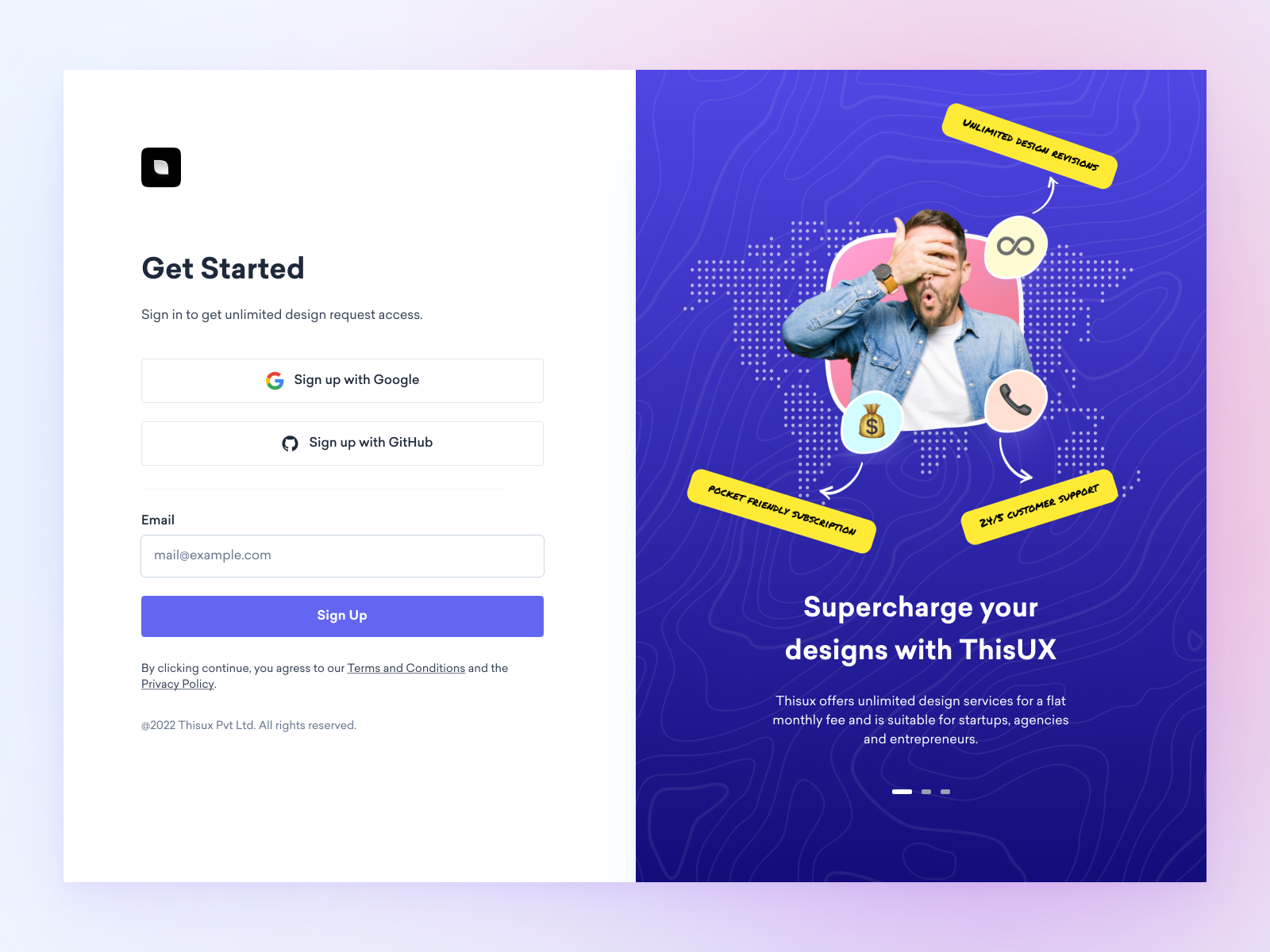The image features a webpage designed for a design request service. In the upper left corner, the text "Get Started" invites users to sign in and gain unlimited access to design requests. A black square with a small diamond icon is positioned at the top, adding a minimalist decorative touch. The background of the page transitions through hues of white, purple, and pink.

The main interactive elements include a clickable "Sign up with Google" rectangle, followed by another option to "Sign up with GitHub." Below these buttons, there is a rectangular field for users to enter their email address. A blue "Sign Up" button is situated towards the bottom of the form. Beneath this button, a disclaimer reads, "By clicking continue, you agree to our terms and conditions and the privacy policy," along with a copyright notice from 2022.

On the right side of the page, a central image features a man with his hand over his eye and his mouth forming an "O," suggesting surprise. The background of this segment displays a dotted map pattern. Text overlays the image, detailing the service offerings: "Unlimited Design Requests," "Pocket-Friendly Subscription," and "24/7 Customer Support." Above the man's head, a headline encourages users to "Supercharge your designs with this U.S.-based service."